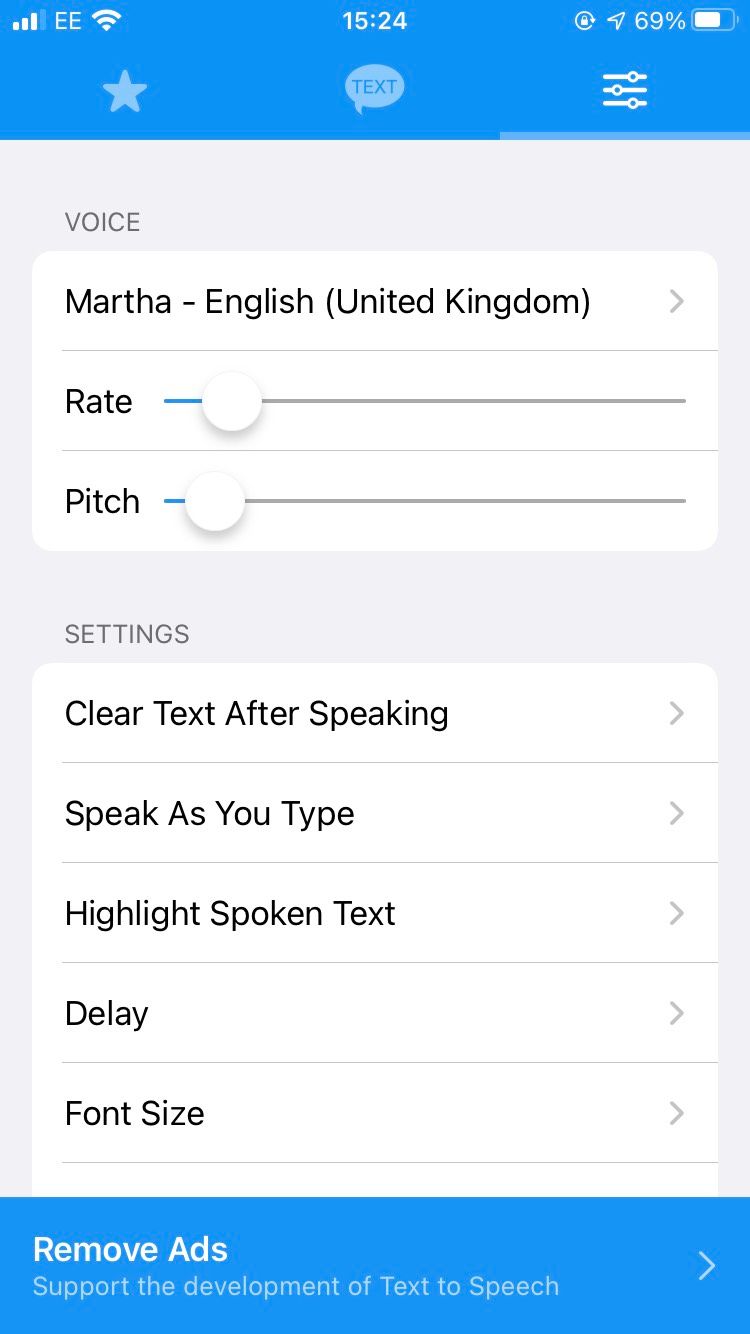This image is a screenshot of a free texting application. The interface is cleanly designed, characterized by a prominent blue header at the top. Embedded within this header, from left to right, are icons for cell signal strength, WiFi connectivity, the current time, location services, and battery percentage.

Underneath the header, still within the blue border, reside three small icons: a star on the left, a text chat bubble in the center, and a settings gear on the right.

The body of the app is predominantly gray. At the very top of this gray section, the word "Voice" is displayed boldly. Directly beneath it is a white settings box that reads "Martha English, United Kingdom," with an arrow indicating the option to change voices.

Further down, there are adjustable slider bars labeled "Rate" and "Pitch," allowing the user to modify the voice settings.

The interface then sections off into a settings category, clearly marked by the word "Settings" in gray at the top left. Below this, another white settings box presents different customizable options:
1. "Clear text after speaking" with an arrow for adjustment.
2. "Speak as you type," also accompanied by an arrow.
3. "Highlight spoken text," again with an arrow.
4. "Delay," providing yet another arrow for modifications, and 
5. "Font size," which likewise has an arrow for adjustments.

Finally, at the bottom of the screenshot, a blue pop-up banner prominently suggests "Remove ads," accompanied by an arrow pointing to the left.